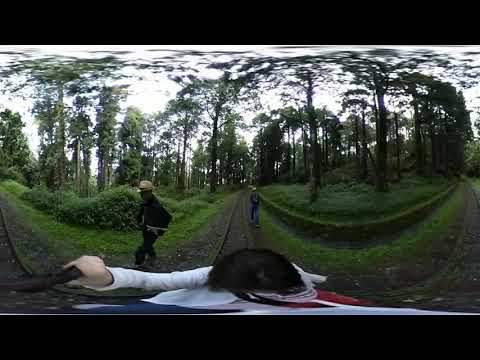The image captures a dynamic outdoor scene on a bright, clear day. The foreground shows a person riding a white mountain or dirt bike, with visible handlebars and a black central piece. The rider's gloved hand is gripping one handle, and part of their outfit is visible, featuring red and blue colors.

To the left, a person dressed in all black is seen, possibly wearing skates or another unclear form of foot gear due to the cutoff at the bottom of the image. This individual has a long-collared shirt covering their mouth, sunglasses, and blonde hair, with a stick positioned across their arms, looking downwards to the left.

In the front right, another person approaches, also possibly on skates, dressed entirely in blue and sporting a large white necklace and blonde hair. Both are heading towards the primary scene of the bike rider.

Further back, on the left and right sides, there are partially blurred tracks made of metal sides, suggesting a pathway, surrounded by trees and well-trimmed hedges forming a wide U shape. Beyond this, green bushes and trees stretch out, creating a lush backdrop. Distortion from a fisheye lens gives the image a rounded, almost surreal twist, with slightly warped perspectives of the clear sky and forested surrounding.